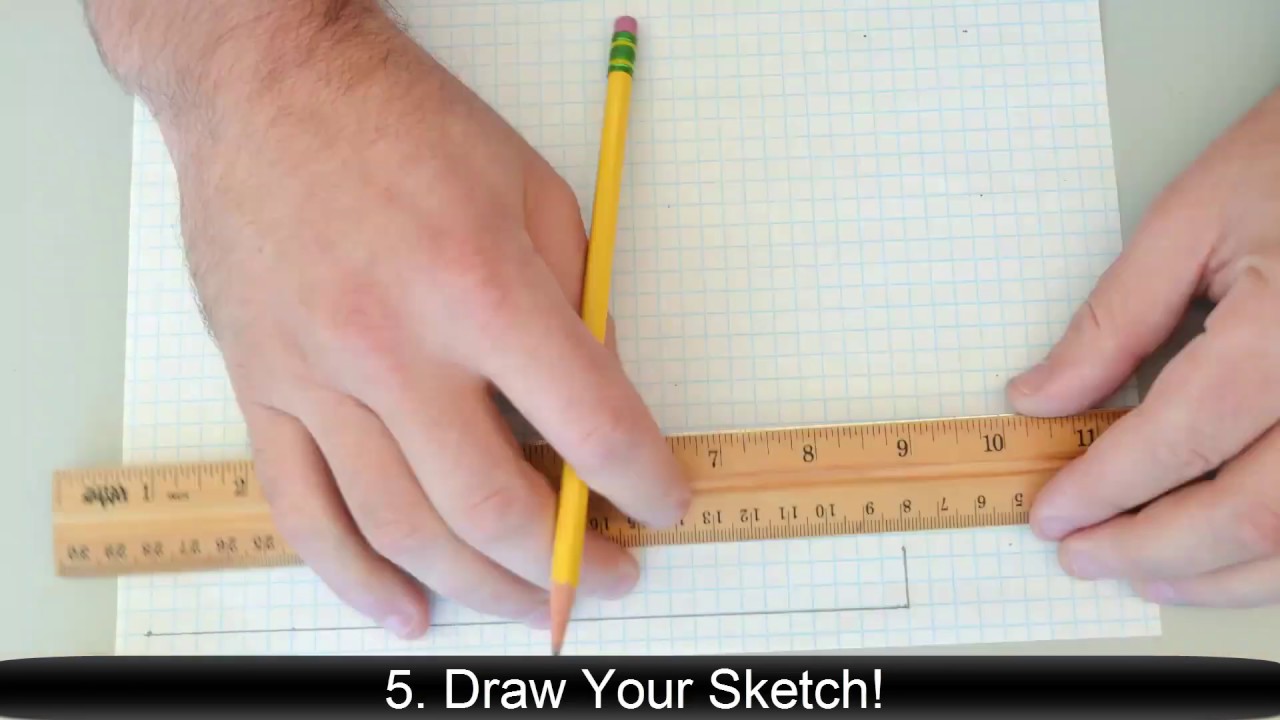In a top-down view, this image appears to be a screenshot from a video, capturing a man's hands as he works meticulously on grid paper with a traditional wooden ruler and a yellow pencil fitted with an eraser. The man's darker body hair is visible on his wrists. He has already drawn two lines on the paper, forming an L shape—one long, horizontal line and one shorter, vertical line—each marked with dots at their endpoints, suggesting a more intricate design in mind. Currently, the ruler is held at an angle that would result in a crooked line if the pencil were to trace along it. Adding to the instructional tone, the bottom of the image features a black banner with the phrase "5. Draw your sketch!" in white block letters, emphasizing its learning context.